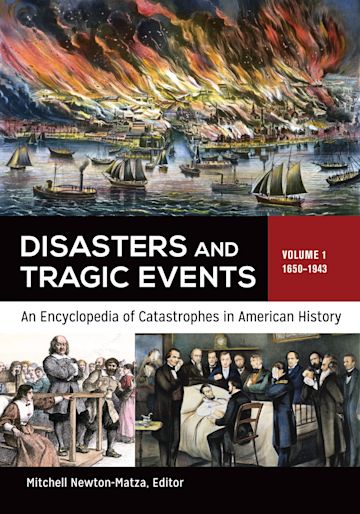This is the front cover of the book titled "Disasters and Tragic Events, Volume 1: 1650-1943, An Encyclopedia of Catastrophes in American History," edited by Mitchell Newton Matzah. The top of the cover features an illustration of a blazing fire engulfing ships in a harbor, possibly depicting an event in Boston, though the exact location is not specified. Below this, the left side of the cover portrays a colonial man in period attire standing in a courtroom-like setting reminiscent of the Salem Witch Trials, with a crowd surrounding him and a young woman in traditional garb seated beside him. The right side shows a solemn scene of Abraham Lincoln on his deathbed, surrounded by several people, including what appears to be his cabinet members and possibly doctors. The cover serves as a visual prelude to the historical catastrophes documented within the book.